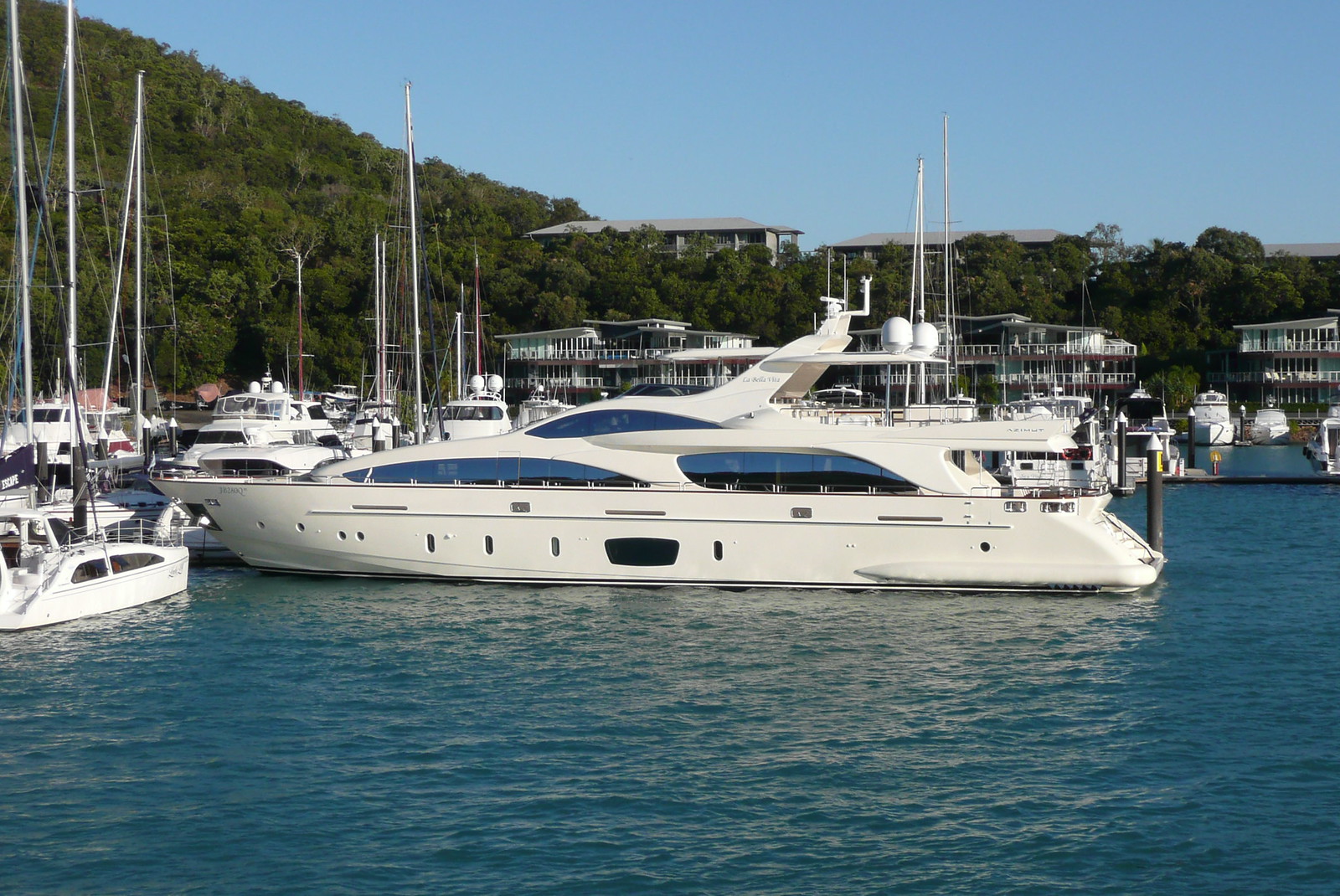In this picturesque harbor scene, a large white and blue yacht dominates the foreground, making an impressive contrast with the smaller sailboats and yachts docked nearby. The yacht, which is the largest vessel in the vicinity, features a sleek design with tiny windows adorned with blue accents, portholes, and a prominent black window area near its base. The yacht's two decks are connected by an elegant staircase, with railings providing safety and a great vantage point for onlookers.

The calm, dark blue water perfectly reflects the yacht and surrounding boats, gently cradling them with its tranquil surface. The backdrop consists of a treed hillside, offering a rich green tapestry that complements the scene. This hillside is dotted with various buildings, including three-story structures with numerous windows and balconies, and possibly shops or restaurants along the shore.

The sky above is a brilliant, cloudless blue, adding to the serene atmosphere of the image. Nestled to the left of the scene is a solid tree line, enhancing the natural beauty of the harbor. In the background, other boats can be seen, including a light green building with white chairs on its decks, further adding to the vibrant and bustling maritime environment. A noticeable figure in a white shirt can be seen on one of these boats, suggesting ongoing activity and life within this peaceful harbor setting.